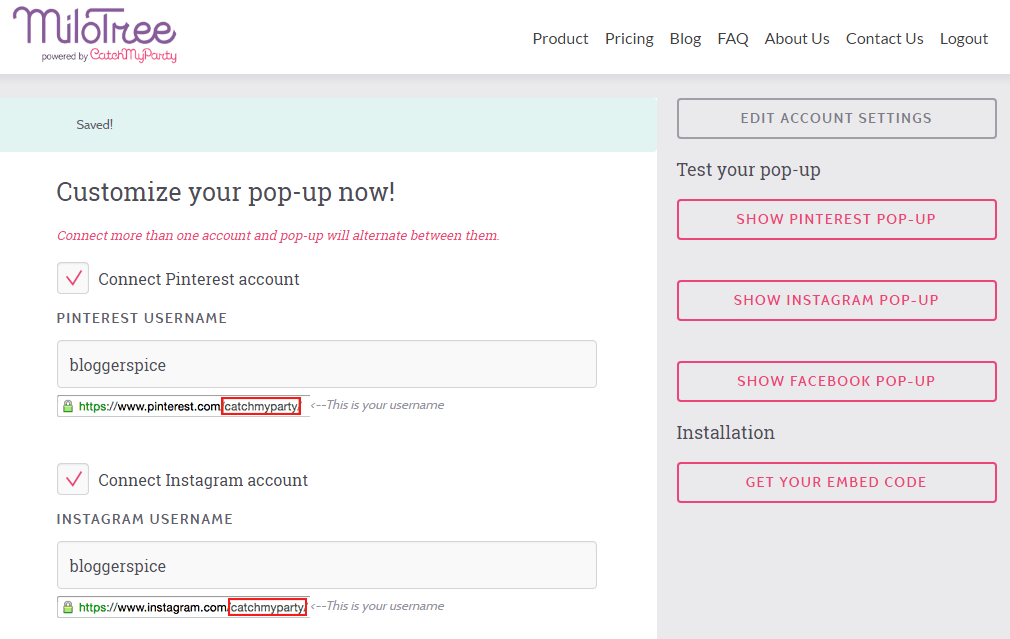**MiloTree App Interface Powered by Catch My Party**

The image showcases the MiloTree app, an interactive tool by Catch My Party. The interface features a vertical menu on the right side of the screen set against a pink background, which seamlessly extends across the top of the page. The menu includes options such as "Edit Account Settings," "Test Your Pop-Up," "Show Pinterest Pop-Up," "Show Instagram Pop-Up," "Show Facebook Pop-Up," "Installation," and "Get Your Embed Code." Each button is delineated with dark pink text or a dark pink rectangular outline, maintaining a uniform size and font. Notably, the "Edit Account Settings" button is distinctly gray.

To the left of the vertical menu, a section with a teal background displays the word "Saved" in bold. Below this, instructions are provided for customizing the pop-up window, connecting multiple accounts, and alternating between them. Adjacent to these instructions is a checkbox with a pink check mark in a gray box indicating the current selections.

Further down, user-specific input fields are present for connecting social media accounts. For connecting a Pinterest account, users are prompted to enter their Pinterest username (e.g., "blogger spice") and the corresponding URL (e.g., www.pinterest.com/catchmyparty). This username field is accompanied by an arrow pointing to "This is your username."

Similarly, for Instagram, users can connect their account by entering their Instagram username and the relevant URL (e.g., instagram.com/catchmyparty). The username "catchmyparty" is highlighted with a pink box for both the Pinterest and Instagram sections for emphasis, although this highlighting appears to be an annotation added post-screenshot and not part of the actual app interface.

This meticulous layout aids in a streamlined user experience, enabling easy navigation and customization within the MiloTree app.